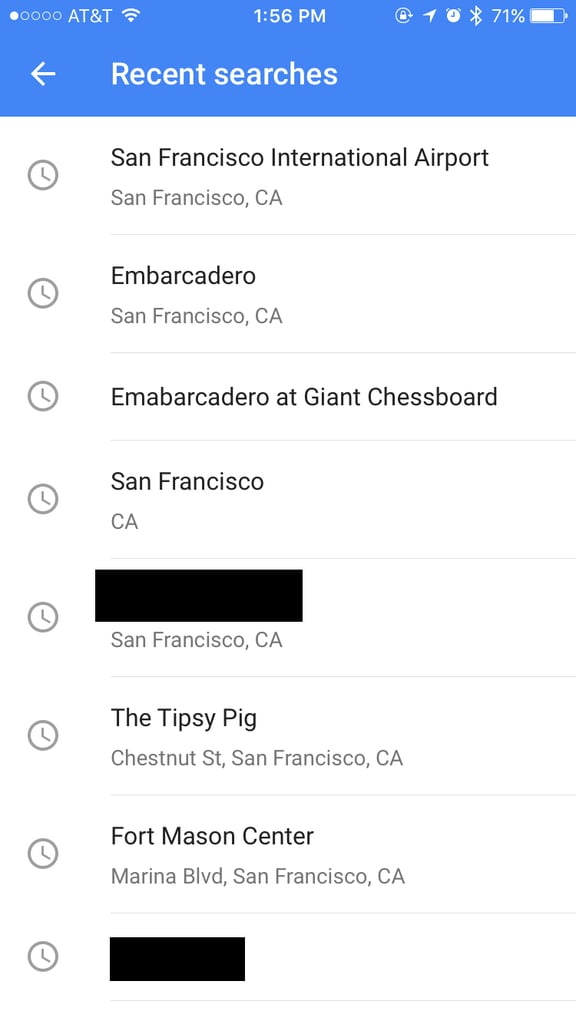Screenshot of a smartphone connected to AT&T with available WiFi. The device displays the time as 1:56 PM and shows a battery level at 71%. At the top of the screen, a blue bar spans horizontally, labeled "Recent Searches" with a left-facing arrow. Below this bar, there is a white background displaying a list of recent search results in black text, including: "San Francisco International Airport, San Francisco, California," "Embarcadero, San Francisco, California," "Embarcadero at Giant Chess Board, San Francisco, California." There are also two entries obscured by black boxes, labeled as "San Francisco, California," and other entries for "The Tipsy Pig, Chestnut Street, San Francisco, California," and "Fort Mason Center, Marina Boulevard, San Francisco, California." Another blacked-out box appears at the bottom of the page.